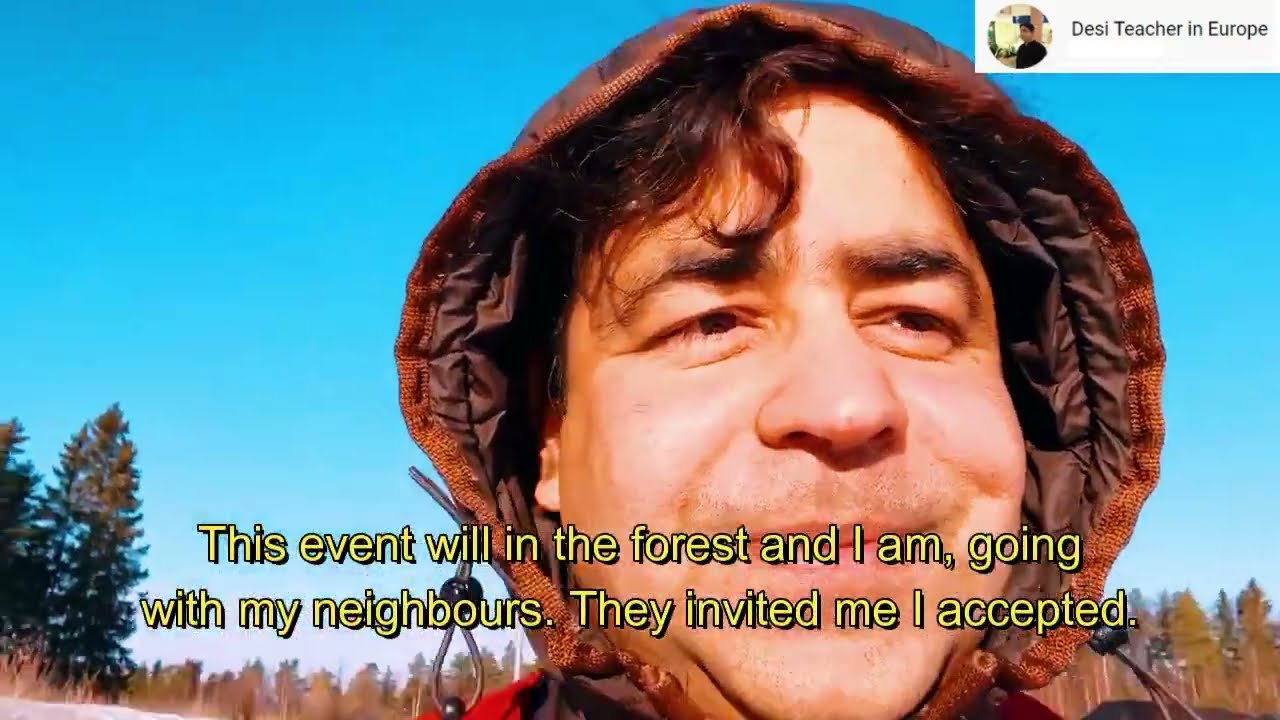The image depicts a medium-skinned man with stubble, wearing a brownish-orange hooded jacket, standing outdoors beneath a vibrant blue sky. His face, shown from just below the chin to the top of his head, displays a smirk and raised eyebrows as if responding to someone off-camera to his left. In the background, a wooded area with pine trees is visible. Overlaying the image are yellow-text captions, reading: "This event will be in the forest and I am going with my neighbors. They invited me. I accepted." In the upper right corner, a pop-up with a channel icon and black text on a white background states, "Desi Teacher in Europe," suggesting that the man might be an Indian teacher residing in Europe.